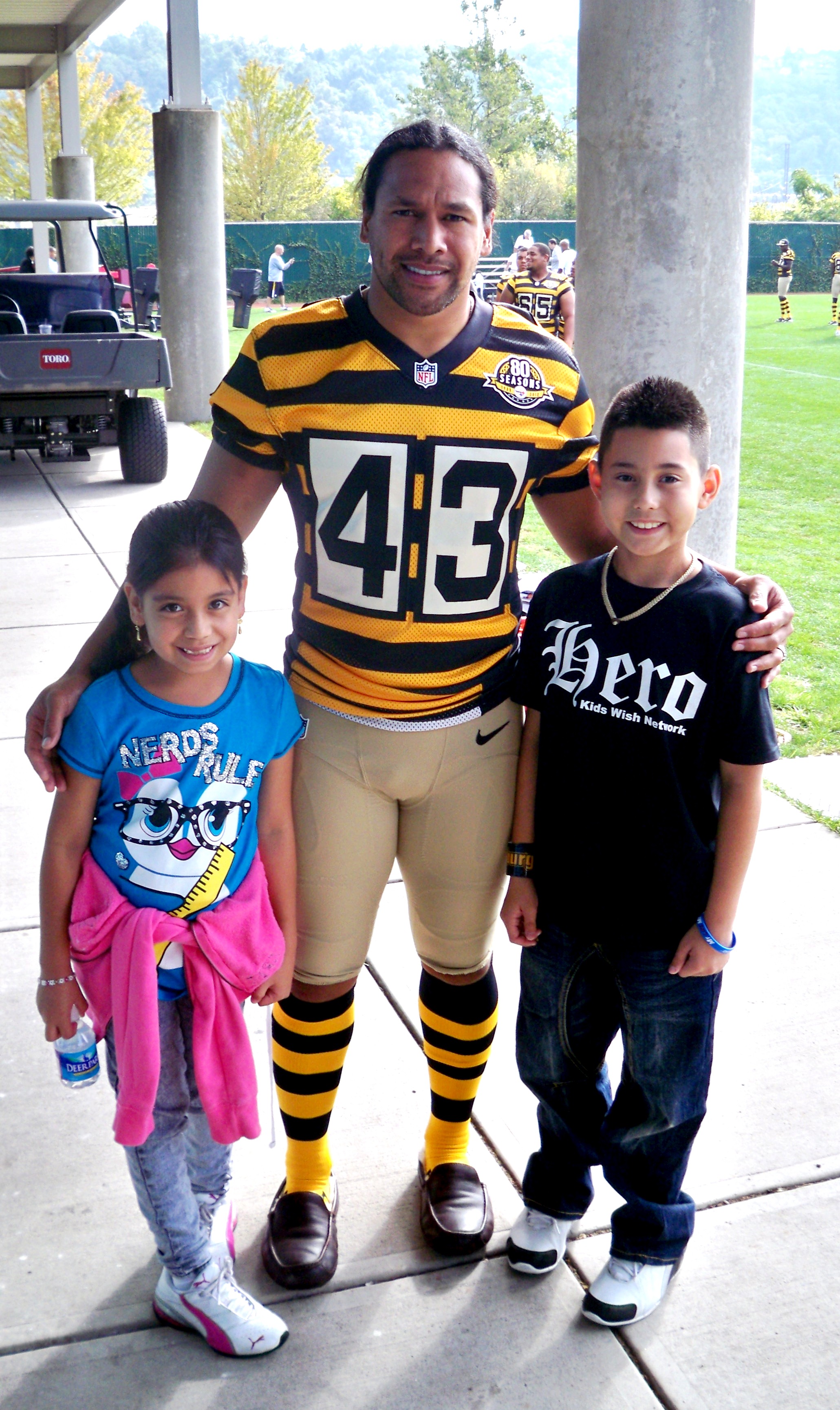The photograph captures a young Latino man standing with two children, posing for the camera. The man, with long dark hair pulled back into a ponytail, is dressed in a yellow and black striped sports jersey featuring the number 43 in bold black numerals on the front, emblazoned on white rectangular backgrounds. His ensemble includes gold knee-length pants with a Nike swoosh near the waist area, black loafers, and black and yellow knee-high striped socks. The jersey also displays an "80 Seasons" patch on the left shoulder and an "NFL" logo in the center.

On his left, the man has his arm around a young girl, possibly around seven years old, who is also Latino with long dark hair. She is wearing a blue t-shirt that bears the text "Nerds Rule" alongside an owl graphic, a pink hoodie tied around her waist, blue jeans, and white shoes. She is holding a bottled water. On his right, his arm rests on the shoulder of a young Latino boy who is wearing a black t-shirt with white lettering that reads "Hero", dark blue jeans, and white and black sneakers.

In the background, other people can be seen, including what appears to be NFL players socializing and practicing on a grass field. The scene is punctuated by a black golf cart parked on a sidewalk to the left, near some pillars of a nearby structure, suggesting an outdoor recreational setting.